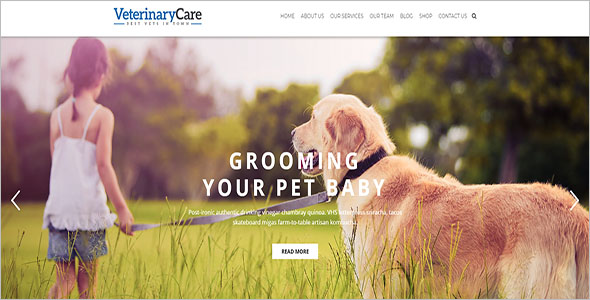The screenshot features a veterinary care website with a sleek and user-friendly interface. Key navigation options, including "Home," "About Us," "Our Services," "Our Team," "Blog," "Shop," and "Contact Us," are prominently displayed at the top, along with a magnifying glass icon for search functionality. The words "Veterinary" in blue and "Care" in black highlight the website's primary focus.

The main image showcases a young girl in shorts and a white shirt walking her brown and white dog with a gray leash. They are outdoors on a grassy area with visible weeds, under a clear blue sky with trees in the background. The headline "Grooming Your Pet Baby" accompanied by additional informative text is prominently featured, encouraging viewers to learn more. Below this, a white rectangle with the prompt "Read More" in black text invites further exploration. Navigation arrows are situated on the left and right sides of the screen, enabling users to browse through additional content. The site’s clean design is further emphasized by a white header at the top.